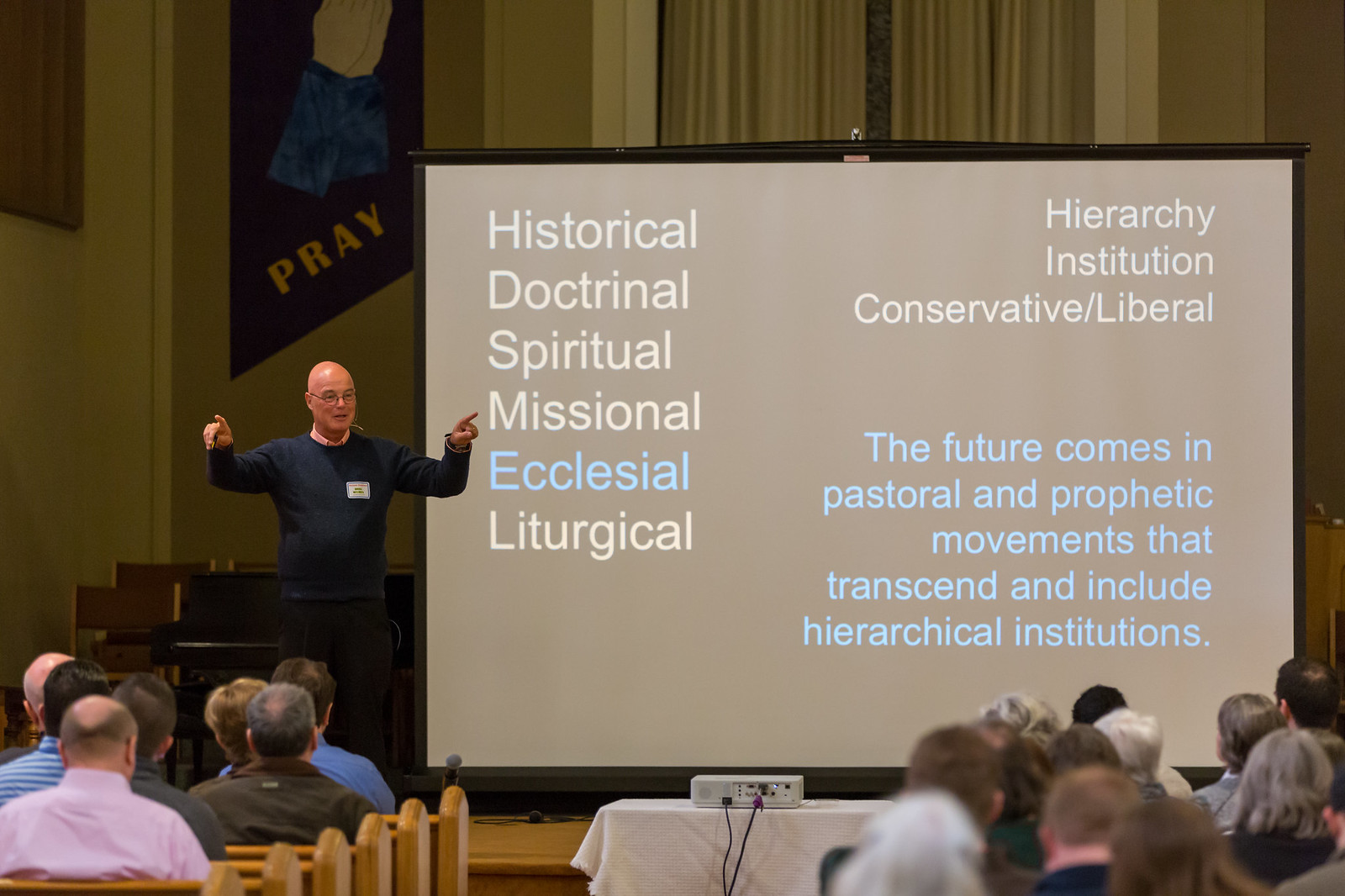In the image, an older white man with a bald head, wearing thin-rimmed glasses, a blue sweater, and black pants, stands on a brown wooden stage in a yellowish-tan walled hall that appears to be a church. He is pointing towards the audience, who are seated in brown wooden pews. Above him, a banner with yellow letters and praying hands reads "Pray." The stage also features a black piano and some brown chairs. A white projector sits on a table with a white tablecloth in front of a large screen. The screen displays text in white and blue fonts: on the left, it reads "Historical, Doctrinal, Spiritual, Missional, Ecclesial, and Liturgical"; on the right, it lists "Hierarchy, Institution, Conservative, Liberal." Below, a phrase reads, "The future comes in pastoral and prophetic movements that transcend and include hierarchical institutions." Curtains hang behind the projection screen, adding to the indoor setting.